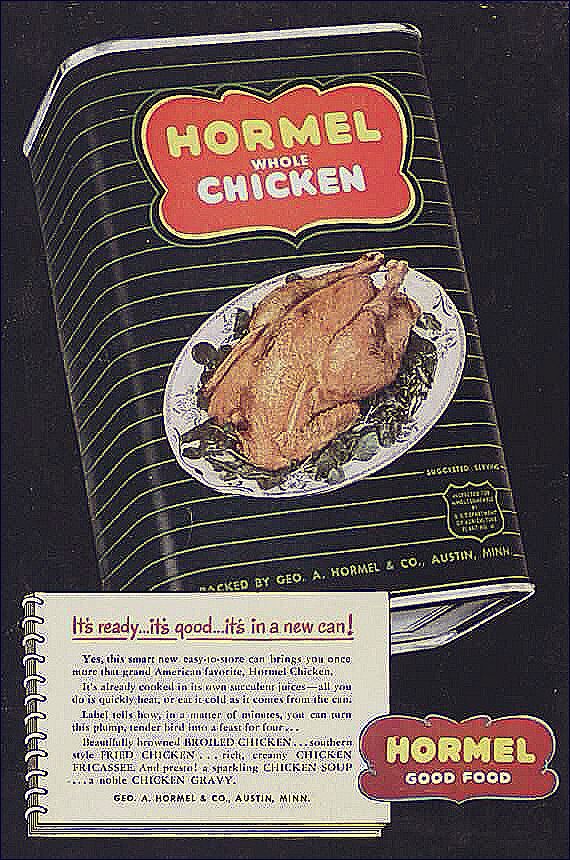This vintage advertisement from the 1960s showcases Hormel's Whole Chicken in a Can. The can, predominantly black with yellow stripes, features an image of a fully cooked chicken resting on a bed of greens, ready to serve. A bold red emblem on the can displays the Hormel logo, with the slogan "Good Food" written beneath. The ad emphasizes the product's convenience and versatility, highlighting that the chicken is already cooked and can be enjoyed either heated or cold straight from the can. The label suggests various dishes you can prepare, such as beautifully browned broiled chicken, southern-style fried chicken, creamy chicken fricassee, hearty chicken soup, and rich, noble chicken gravy. Additional text describes the chicken as being plump and tender, stored in its succulent juices, making it a practical meal solution. Produced by Hormel Company in Austin, Minnesota, this product embodies the brand's promise of quality and convenience.